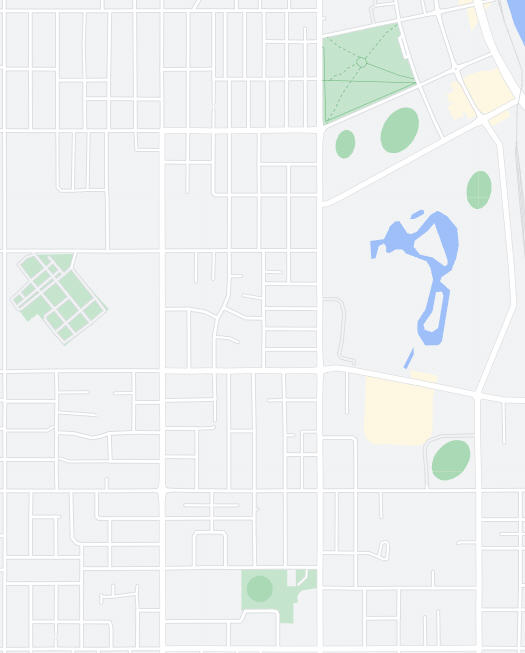This image is a Google Maps screenshot showcasing an urban area designed in a grid layout. The screenshot is devoid of granular details such as housing structures, road textures, business locations, or street names. The map primarily highlights the streets and their connections, allowing one to navigate based on directional pathways rather than specific landmarks. To the top right of the image, there's a noticeable body of water, and another smaller body of water is slightly below and to the left. Sparse patches of greenery are interspersed among the tightly woven streets. This simplified map provides a high-level view of the area, focusing solely on the network of roads and their intersections without any additional contextual or identifying features.